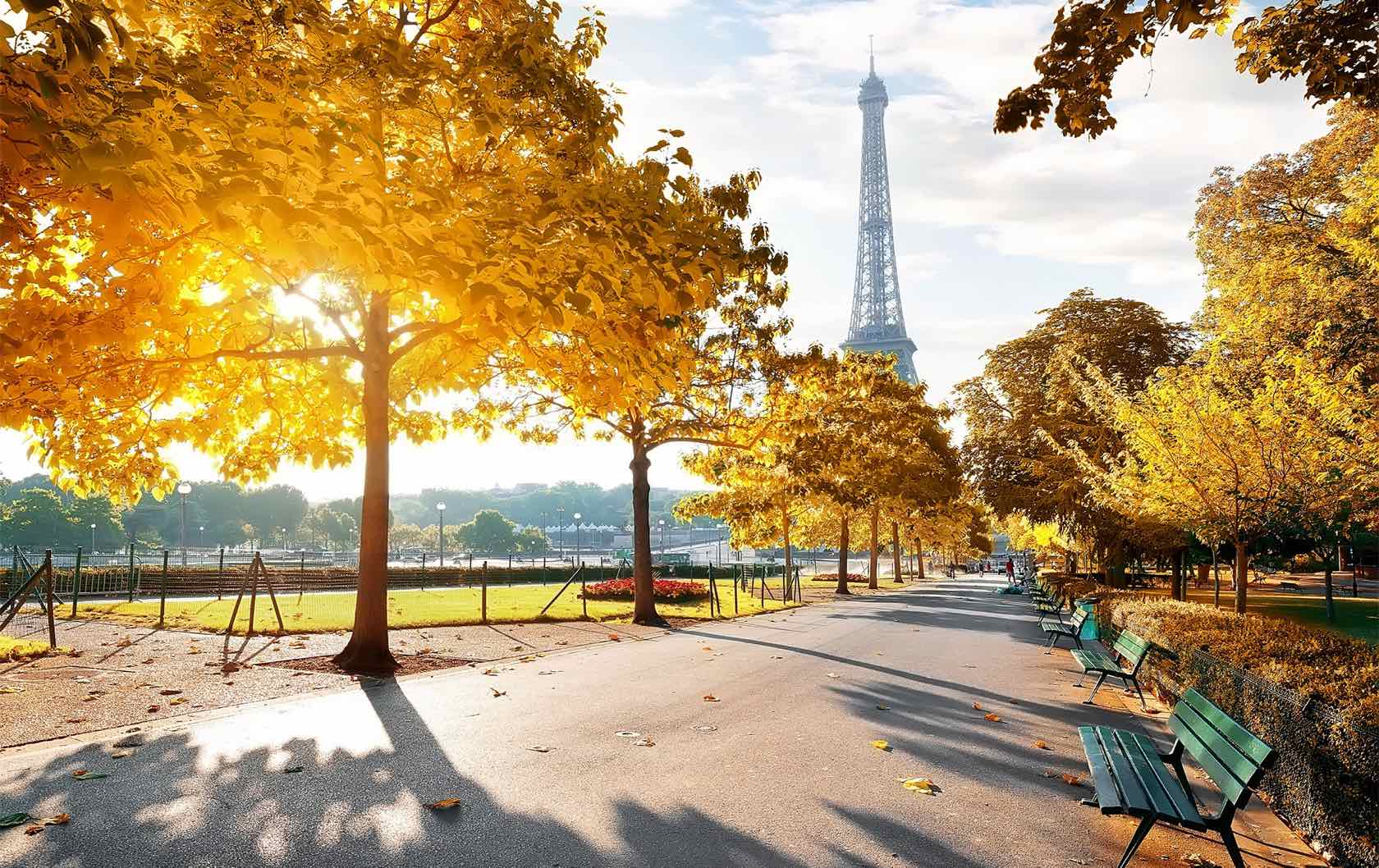This vividly lit image captures a picturesque park in Paris during the fall, with the iconic Eiffel Tower in the distant background. The wide pedestrian pathway, positioned centrally, is flanked by trees adorned with vibrant orange leaves and interspersed with other trees sporting yellow and green foliage, all aglow in the sunlight. Scattered leaves blanket parts of the pathway, adding to the autumnal charm. Green benches dot the path, inviting pedestrians to sit and enjoy the serene surroundings. On the right side, the park features a grassy area with mulch surrounding the tree bases, accented by orange bushes and a flowerbed bursting with red flowers. The clear blue sky with white clouds bathes the entire scene in a warm, inviting light, creating a tranquil setting at the center bottom of the frame, while the Eiffel Tower majestically rises towards the center top, completing the enchanting Parisian landscape.